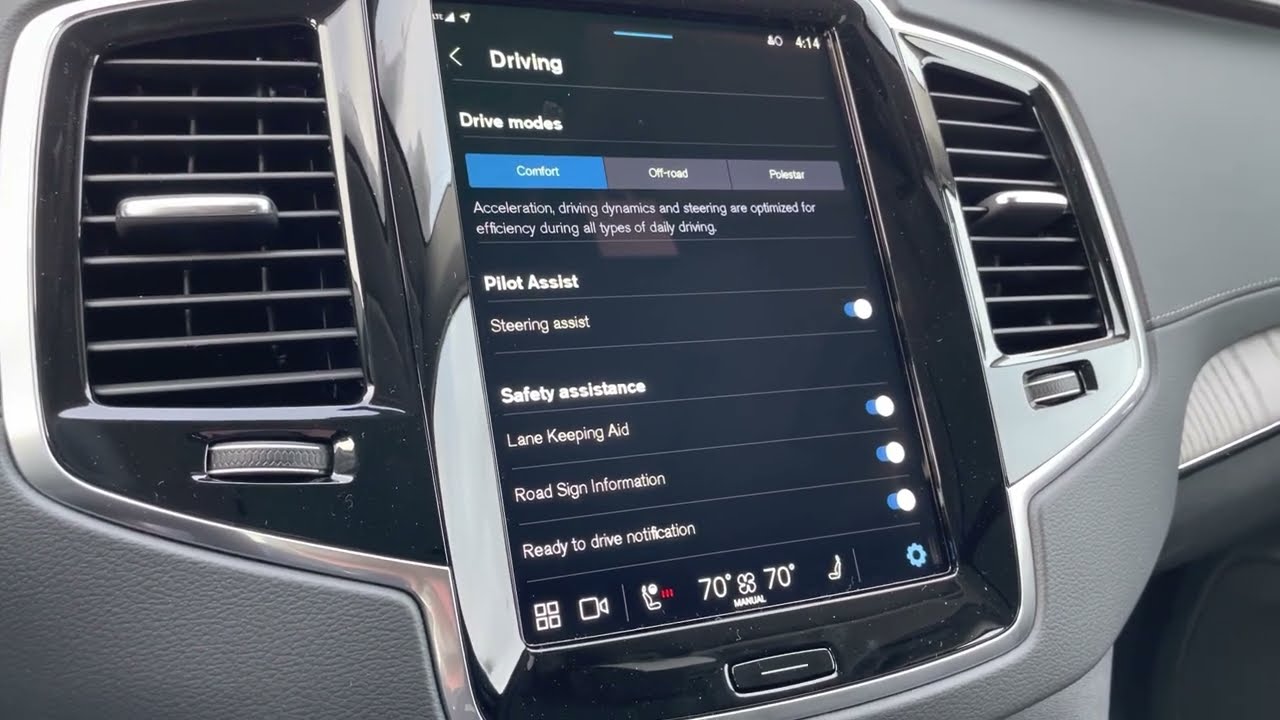The image depicts a close-up photograph of a vehicle’s dashboard focusing on the touchscreen interface positioned at the center. The touchscreen, with a black background, prominently displays a menu under a section titled "DRIVING" located at the top left corner. Adjacent to this title is a left-pointing triangular arrow. On the upper right corner of the screen, the time is shown as 4:14. Below "DRIVING," the menu lists "DRIVE MODES" featuring three options: "COMFORT" in a blue rectangle, "OFF ROAD," and "POLESTAR" in gray rectangles. Further down, the descriptions "acceleration, driving dynamics, and steering are optimized for efficiency during all types of daily driving" are noted. Beneath this description, the screen shows options for "PILOT ASSIST," including "steering assist," "safety assistance," "lane keeping aid," "road sign information," and a "ready to drive notification." All these features appear to be activated. Surrounding the screen are two air conditioning vents equipped with silver partitions and adjustment wheels. The vehicle's interior is gray, and on the lower portion of the touchscreen, the temperature is indicated as 70 degrees, along with a gear settings icon on the bottom right.